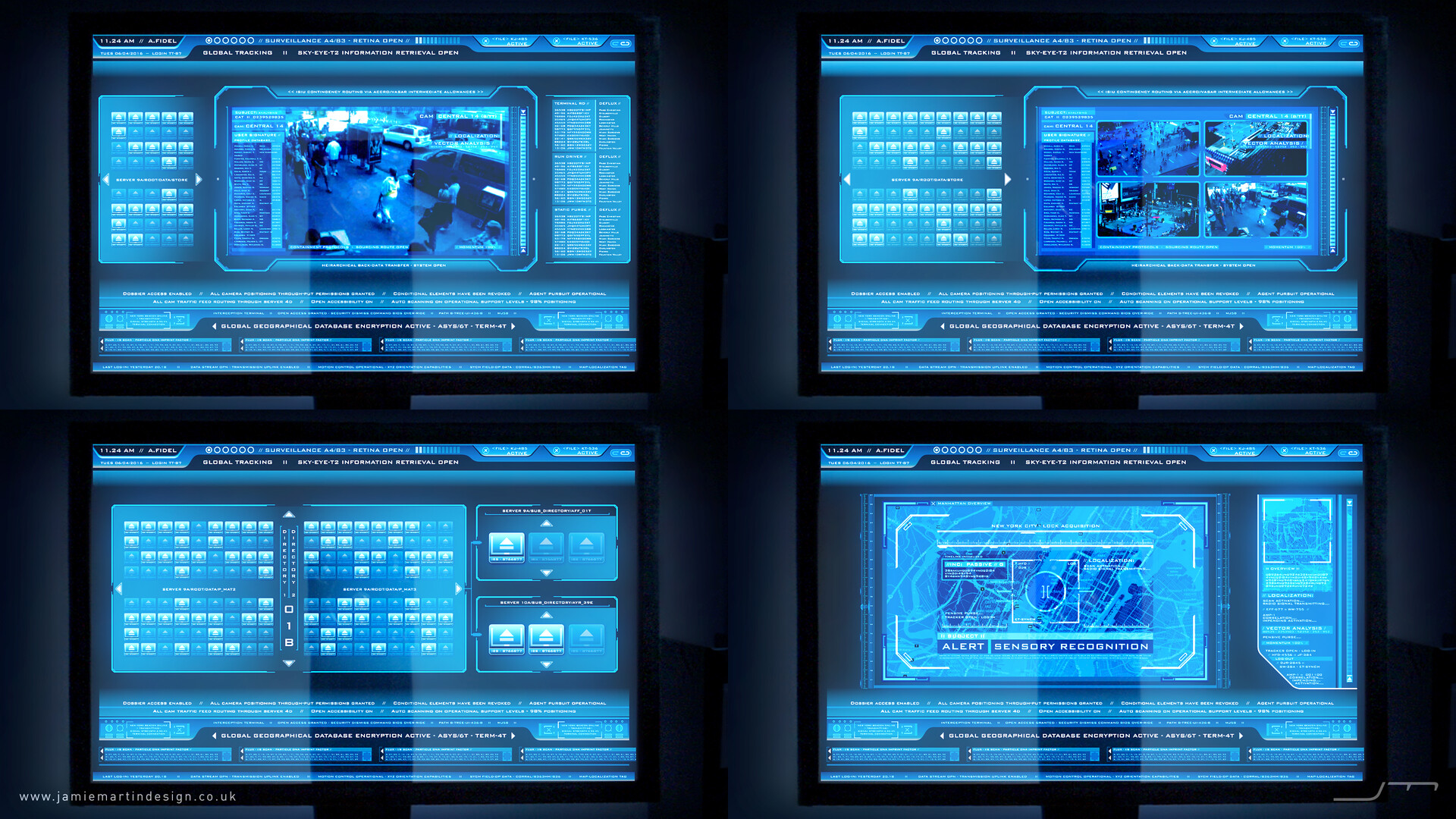The image features four distinct computer screens set against a dark blue, nearly black background, each with a bluish hue. The top left screen shows security camera footage of a bustling main street with several pedestrians commuting on the sidewalk and multiple cars passing by. The top right screen displays additional surveillance images capturing similar street activity, with people walking and vehicles in motion. In the bottom left screen, the display is filled with a series of categorized boxes and buttons, resembling a technical layout or keyboard, though specific details are unclear. The bottom right screen features an alert system interface with the text "alert sensory recognition," possibly indicating a triggered alarm. Collectively, the screens suggest a sophisticated security monitoring and alert system.